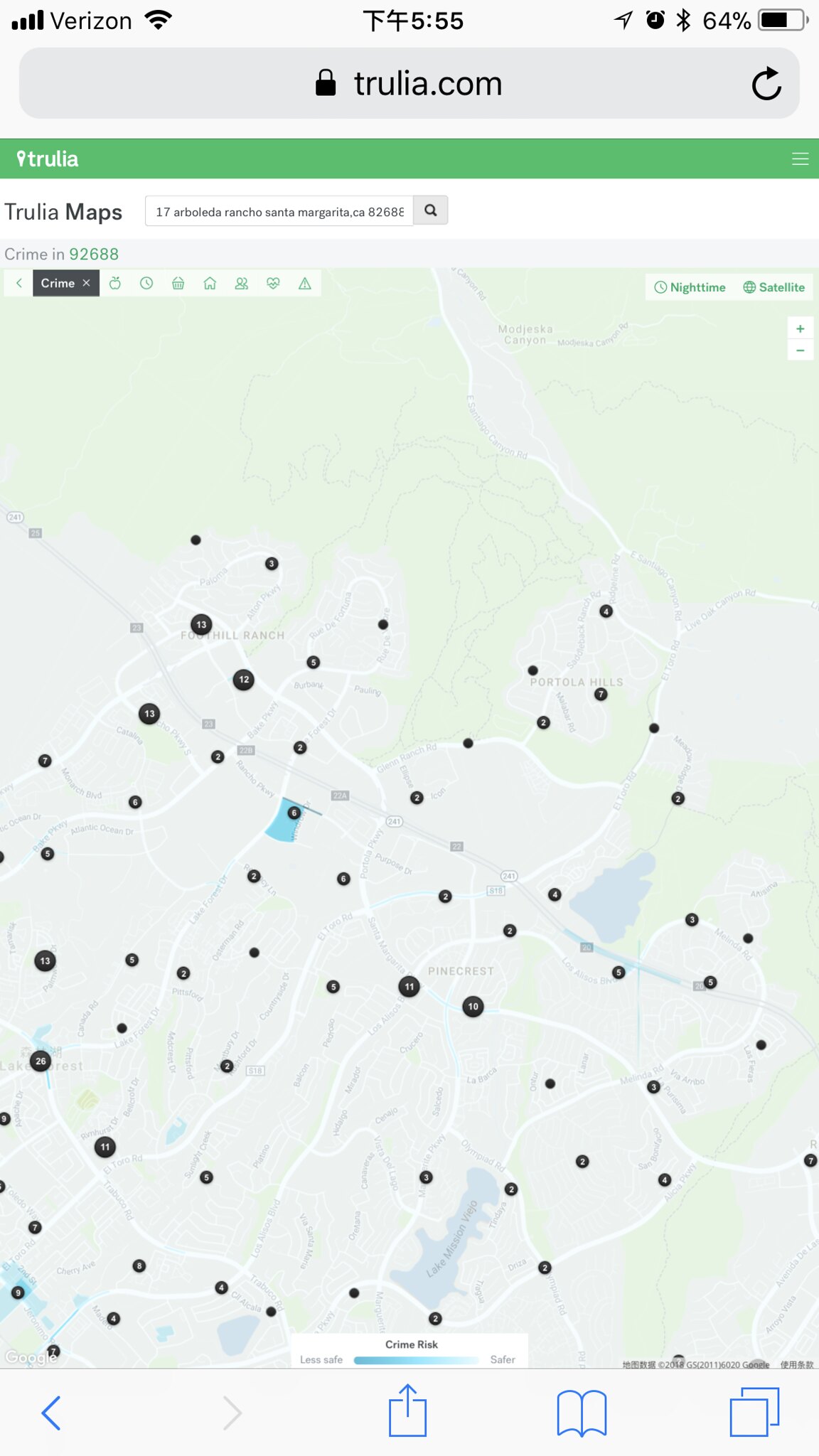This image is a screenshot of search results from Trulia Maps on Trulia.com. The search bar contains a residential address, though the text is too small to be legible. The address appears to be located in California. The map features a pale gray background with very faint green areas indicating possible forests and several pale blue patches representing lakes. A prominent highway runs diagonally across the map, intersecting with numerous white side roads that resemble country roads, suggesting a rural setting. The map is dotted with multiple black markers, which likely indicate the locations of various homes or businesses. A bold turquoise flag highlights the specific residence being searched. At the top of the page, a green banner displays the Trulia logo on the left in white. To the right of the banner, information about crime statistics in the zip code 92688 is provided.